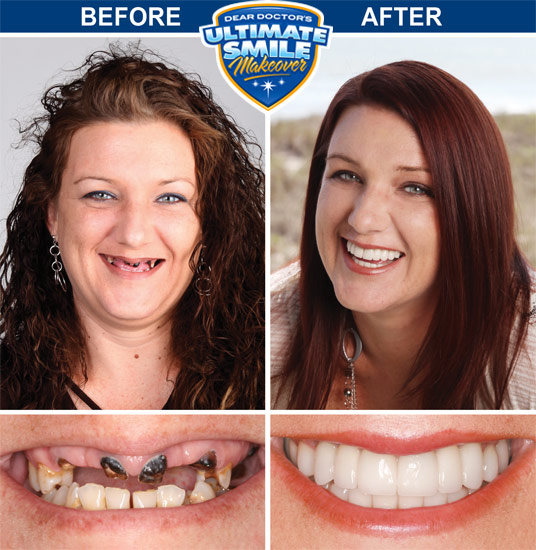The image is an advertisement for dental work with the title "Dear Doctor's Ultimate Smile Makeover" prominently displayed in a shield at the top center, flanked by a large blue bar that labels the left side "Before" and the right side "After." On the left is a frontal photo of a burgundy-haired woman with unkempt, curly hair, smiling to reveal severely decayed and missing front teeth. Directly below this is a close-up of her rotting teeth, emphasizing their poor condition. In contrast, the right side shows the same woman post-makeover, now almost unrecognizable with straight, well-kept hair and a radiant smile. A close-up below this image highlights her new, flawless white teeth, underscoring the dramatic transformation.